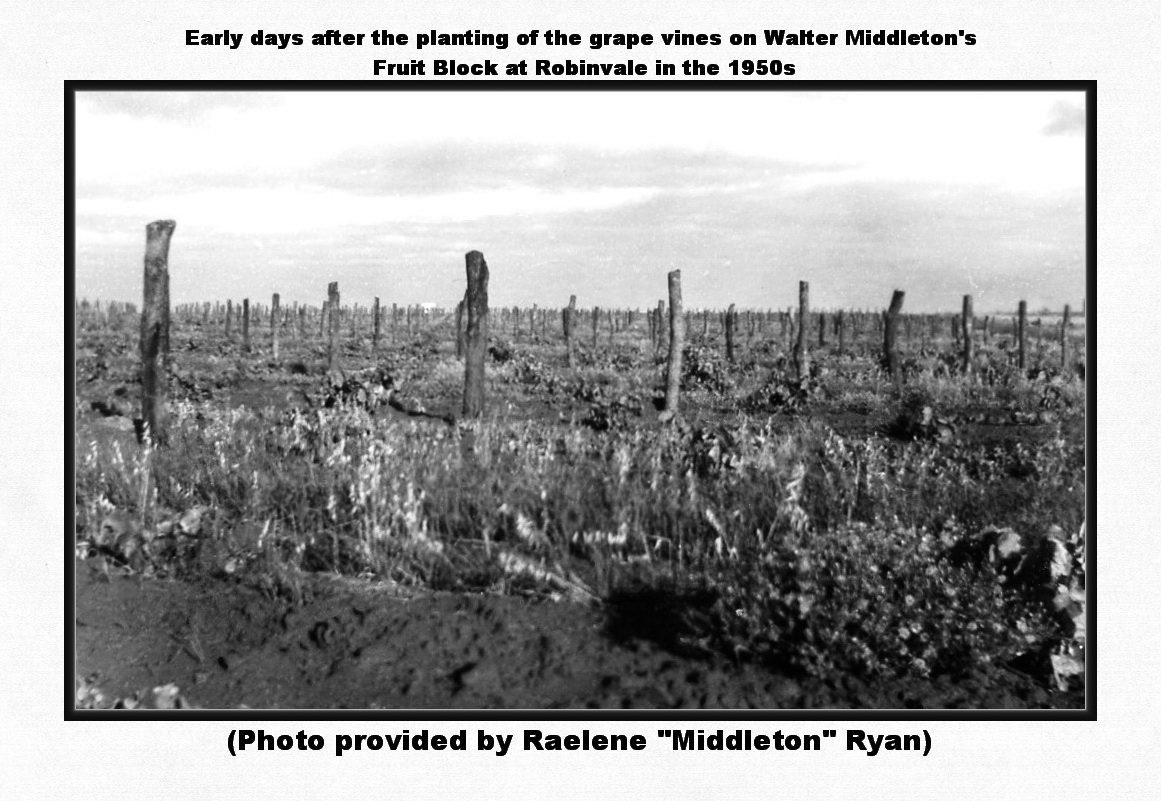The image is a black and white photograph capturing a desolate farm scene, possibly in the fall or winter of the 1950s. The photograph is not in sharp focus, adding to its aged look. The top of the image bears the caption, "Early days after the planting of the grapevines on Walter Middleton's fruit block at Robinvale in the 1950s." Below the photograph, another caption reads, "Photo provided by Raylene Middleton Ryan." The landscape shows a field filled with numerous log poles or stakes, possibly grapevines in their early stages of growth, with no leaves or canopy. Some bushes are visible in the foreground along with disturbed dirt. The sky above is covered with dark, grayish clouds, creating a somber atmosphere as though it might rain. The overall quality of the image reflects the photographic limitations of the time, making the details somewhat difficult to discern.